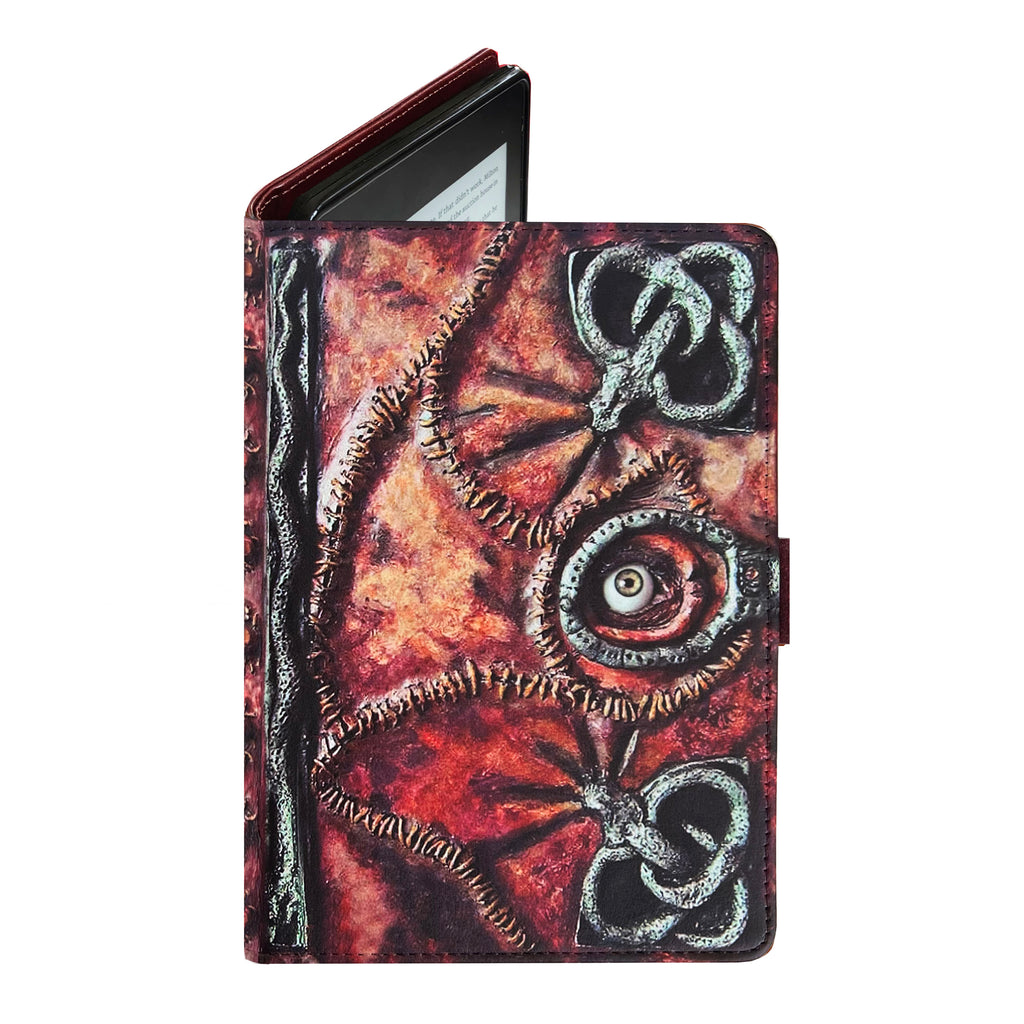This image depicts a very eerie cover designed for a Kindle or tablet device, distinguished by its unsettling aesthetic and horror-themed elements. The outer surface resembles red and yellow flesh that appears stitched together, evoking a look reminiscent of "Texas Chainsaw Massacre." The cover has a black binding that adds to its macabre appearance. Prominent on the cover are circular designs featuring three interlocking rings, which resemble a snake coiling to form the pattern. One of the most striking details is the circular closure tab adorned with a decorative eye, possibly yellow or hazel, giving the impression that it's gazing through a hole in the cover. Additional accents include what seem to be scars with stitches running through them and possibly tentacle-like shapes or a bug. This cover, with its horror genre cues, seems tailored for enthusiasts of creepy designs, making a bold statement that could befit a horror fan's collection.